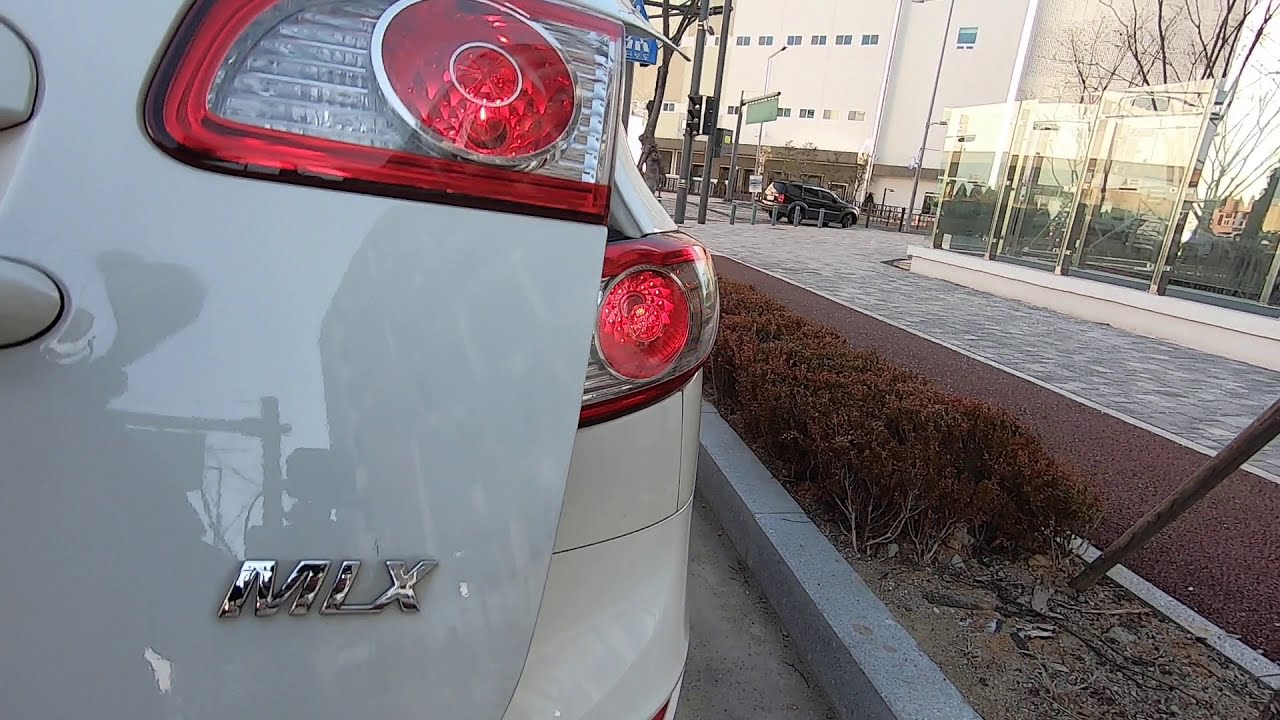This image prominently features the back end of a car, particularly zoomed in on the left half. The vehicle is an icy green color and prominently displays a silver badge reading "MLX." The taillights, combining red and silver, are visible alongside the trunk, which appears slightly opened. The car is parked adjacent to a curb, with a small median of brown, dying plants and low bushes separating the road from a cobblestone pedestrian walkway.

To the right of the car, stretches the pedestrian path that leads past various buildings, one notably featuring entirely glass sides, possibly indicating an entrance to a subway or office complex. In the farther background, a large building appears, accompanied by another black minivan parked near it. Distant streetlights and a few indistinct signs—one green and one blue—are visible, and there seems to be a person standing far away. The overall scene captures a slice of urban environment with a focus on the parked car and its surroundings.